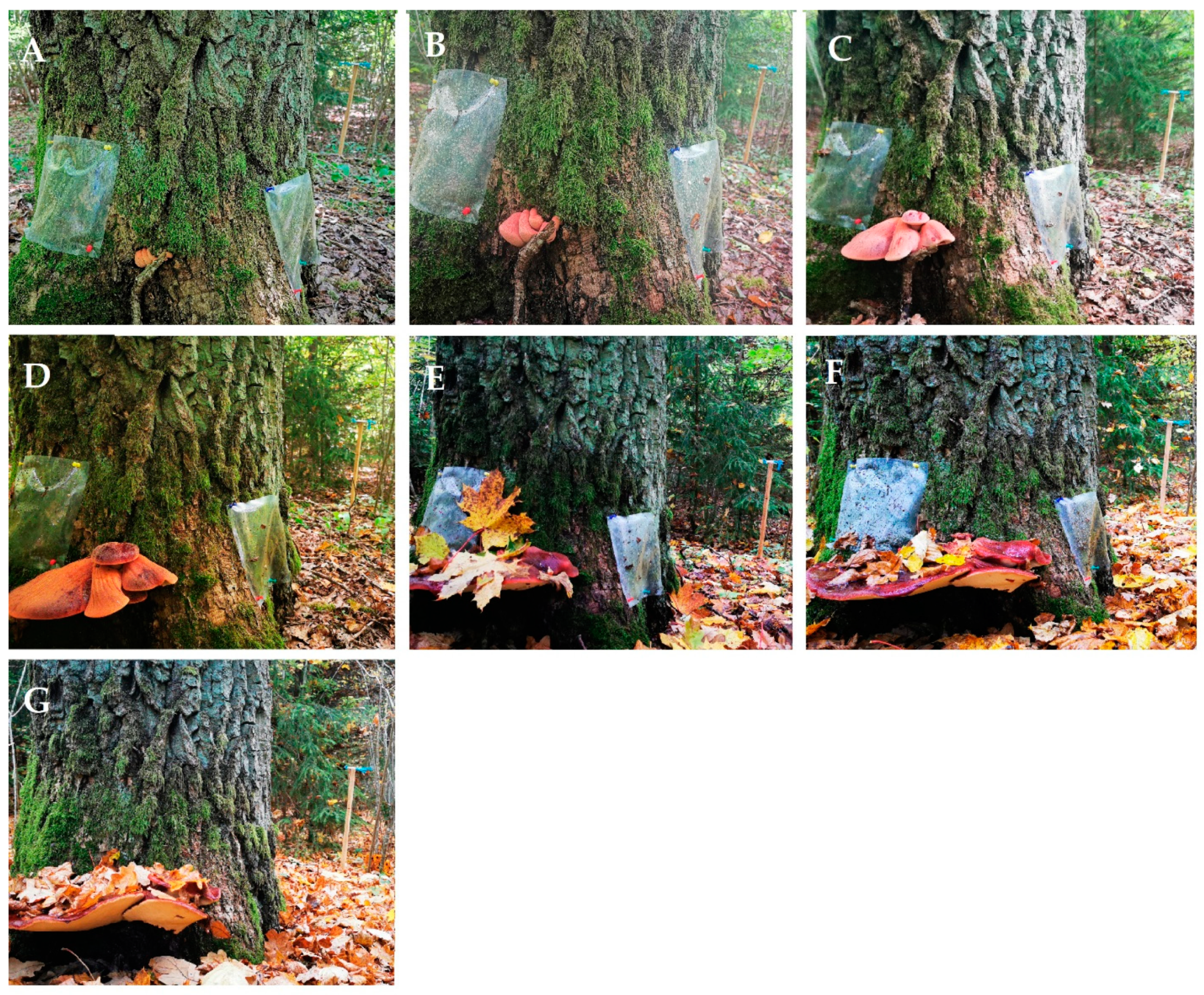The multi-pane photograph series (labeled A through G) captures a progressive outdoor scene centered around an oak tree trunk adorned with bracket fungi and other natural elements. The series consists of seven images, arranged in three rows (three cells in the top row, three in the second row, and one in the third row).

In panel A, the oak tree displays lush green moss at its base, alongside small plastic labels pinned with push pins. A tiny red growth, initially indiscernible, appears on the tree bark. As the sequence advances to panel B, the red form has noticeably expanded.

By panel C, the red growth further enlarges, suggesting the development of a mushroom-like structure. Panel D shows the form becoming noticeably wider with a more pronounced red-orange hue. In panel E, this growth now resembles a shelf fungus, adorned with an arrangement of autumnal leaves in vibrant reds, oranges, yellows, and greens.

In panel F, the fungus broadens even more, accentuating its resemblance to a natural shelf, continuing to support various leaves and decorative elements. The final panel, G, illustrates the underside of the fungi curling upwards, revealing an intricate yellow-orange texture beneath. Throughout the panels, the forest floor beneath the tree gradually accumulates more fallen leaves, culminating in a dense carpet of autumn foliage in the last image. The reflective surfaces and the systematic arrangement imply not just an organic growth but also a creative instructional display for organizing natural elements on tree bark.